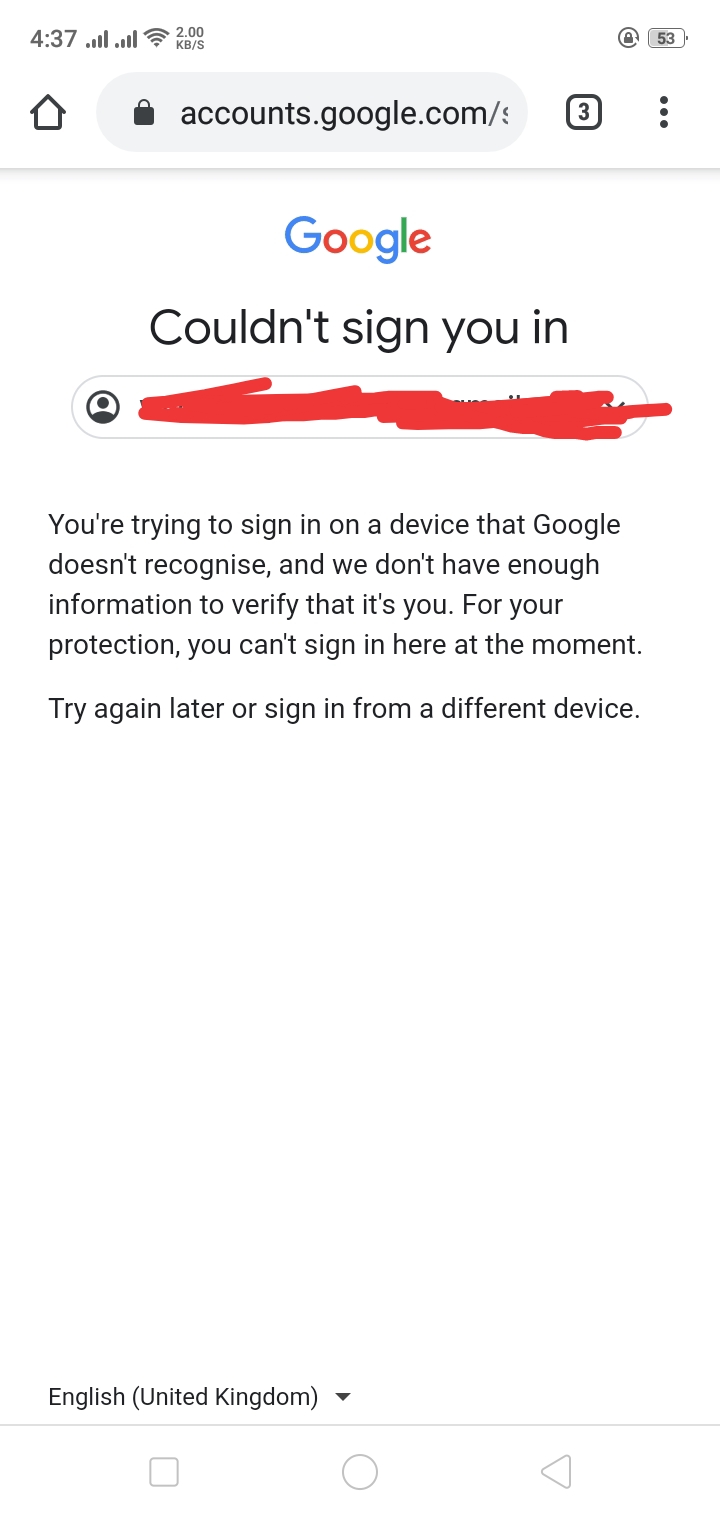The image is a screenshot taken from a smartphone. In the upper-left corner, the time is displayed as 4:37, while the upper-right corner shows the battery icon. Below this, within an oval-shaped box, the URL "accounts.google.com" is visible, and underneath that, the word "Google" is written in its characteristic colorful letters. The main text on the screen states, "Couldn't sign you in," followed by a message explaining that the user is trying to sign in on a device that Google doesn't recognize and lacks sufficient information to verify their identity. Consequently, Google has temporarily blocked the sign-in attempt for the user's protection, advising them to try again later or use a different device.

A significant section of the message includes another long oval, where some text has been crossed out in red, making it unreadable. Following this, the screen features a large white space with no additional content. At the very bottom of the image, there is black text reading "English (United Kingdom)" next to a downward-pointing black triangle. Below this, a line separates the bottom section, which contains three gray symbols: a square on the left, a circle in the middle, and a left-pointing triangle on the right.